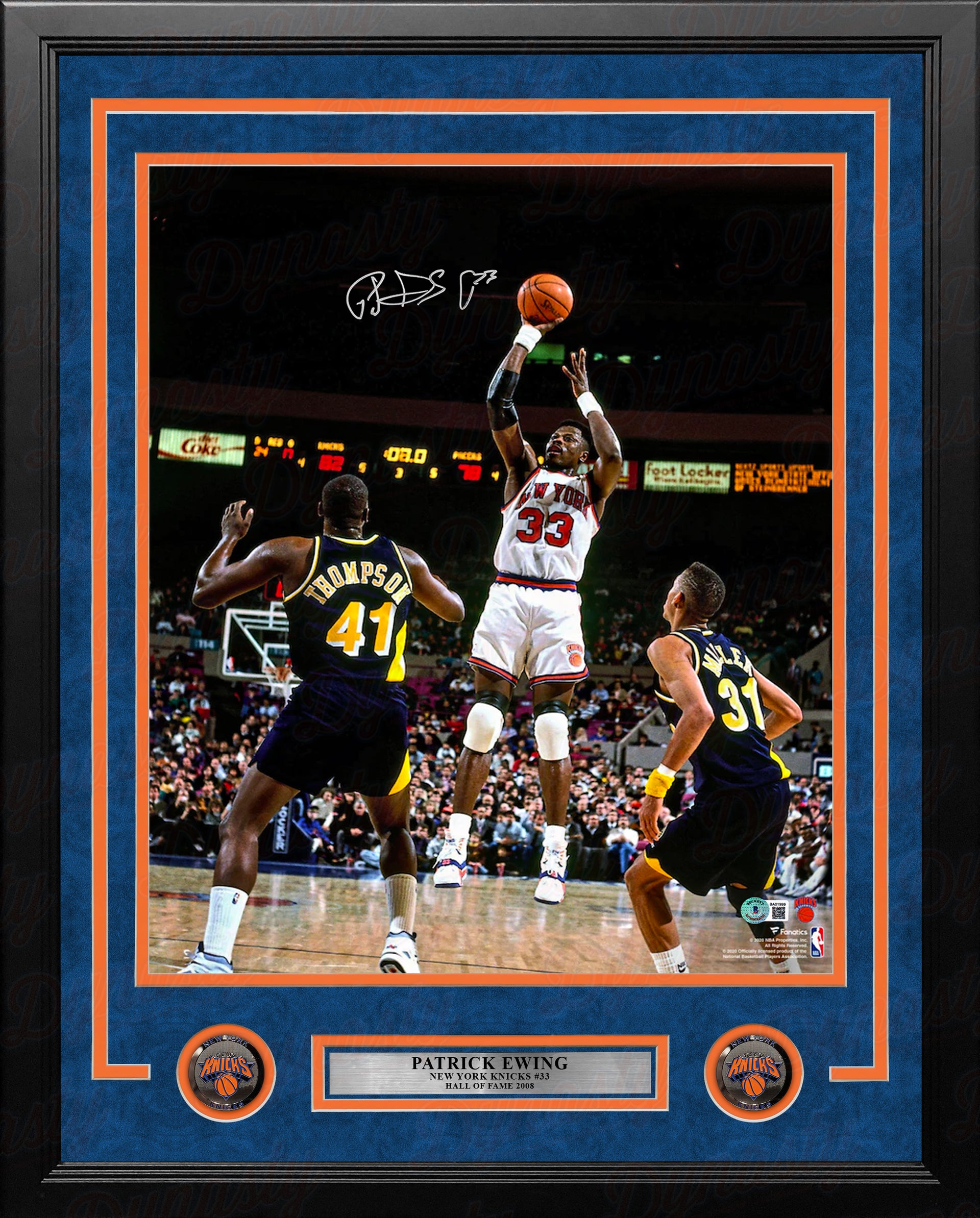This image features a detailed, framed, autographed poster of basketball legend Patrick Ewing. The frame itself is a black vertical rectangle, enclosing a visually striking blue poster with orange trim. At the bottom of the frame, two orange circles with New York Knicks logos flank a horizontal silver nameplate, inscribed in black with "Patrick Ewing, New York Knicks, number 33, Hall of Fame, 2008." The nameplate is outlined by a blue and orange border.

Dominating the frame is a large vertical photograph of Patrick Ewing in action. Ewing, sporting the number 33, is captured mid-jump shot, facing the camera with his right arm extended. He is donning a white jersey and pants with red lettering that reads "New York." His uniform is complemented by white knee pads and white high-top sneakers. Above him, to the left, near the ball, is his silver autograph, which reads "Patrick Ewing #33."

In the foreground, two Indiana Pacers defenders watch Ewing's shot intently. The players, identified by their dark blue jerseys with yellow text, are Thompson, number 41, and Reggie Miller, number 31. The packed stands of the basketball court provide a dynamic backdrop to this high-energy moment. This expertly framed poster, with its vivid colors and detailed inscriptions, celebrates Patrick Ewing's illustrious career and his induction into the Hall of Fame in 2008.